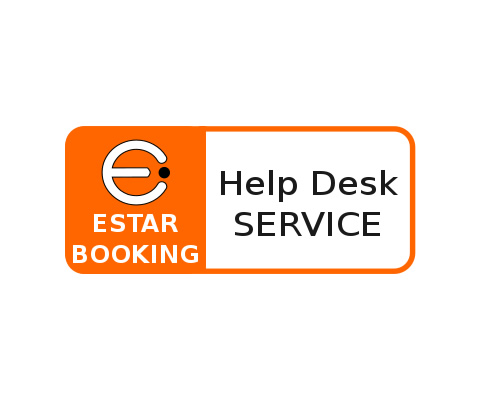The image is a detailed logo for a business named E-Star Booking, designed with a rounded-edge rectangular shape. The left third of the rectangle features a solid orange background that contains the company's logo, which is a stylized white "E" resembling a euro sign, accompanied by a small black dot. Below the emblem, in white text, it reads "E-Star Booking" with "E-Star" on one line and "Booking" directly beneath it. The remaining two-thirds of the rectangle is outlined in orange and has a white interior. Within this white section, the words "Help Desk Service" are prominently displayed in black font, with "Service" capitalized. The entire design resembles a keychain tag and serves to advertise that E-Star Booking offers some form of IT Help Desk service, although the exact nature of the business remains somewhat unclear. The image is crafted in a landscape orientation with a clean and modern infographic typography style.